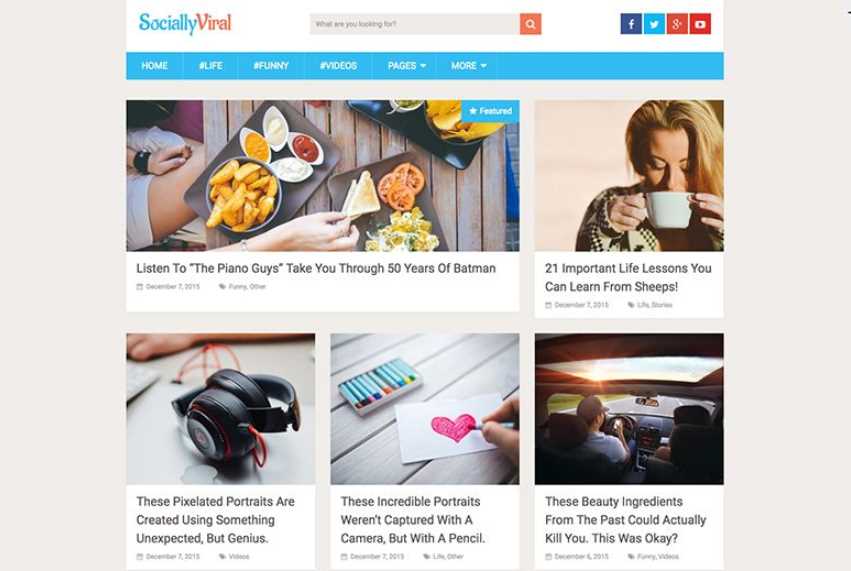This detailed caption describes a screenshot taken from a website, focusing on both the layout and the content presented within the screenshot.

At the upper left corner, "Socially Viral" is prominently displayed in blue and red text. The website's interface includes two light grey bars on both the left and right sides. Adjacent to the "Socially Viral" logo, there is a search box flanked by various social media icons, including Facebook. A blue navigation bar, featuring white text, lists menu options such as "Home," "About," and "Money." Small, unreadable writing is also present, as well as links to "Pages" and "More."

The central area showcases diverse images. Notably, there is an enticing picture of food featuring eggs, chips, pasta, and pizza. Below this image, a caption states, "Listen to The Piano Guys take you through 50 years of Batman," which indeed confirms the theme as "50 years of Batman" upon closer inspection.

To the right, a striking image of a woman with long blonde hair drinking from a cup is accompanied by a headline that suggests, "20 important life lessons you can learn from sheep" (notably miswritten as "sheeps"). Further down, in the right-hand corner, an image displays a person's hand with headphones. The accompanying text reads, "These pixelated portraits are created using something unexpected but genius."

Additionally, a photograph captures a hand drawing a pink heart with crayons on a white piece of paper. The caption notes, "These incredible portraits weren't captured with a camera but with a pencil."

Another section shows the interior of a vehicle: a man driving on the left and a woman with long dark hair on the right. The scenery includes a sunset to the left and a grassy landscape with a mountain to the right. The text here warns, "These beauty ingredients from the past could actually kill you."

Overall, the screenshot provides an eclectic mixture of visual and textual content, presenting information ranging from culinary delights and artistry to life lessons and historical beauty tips.